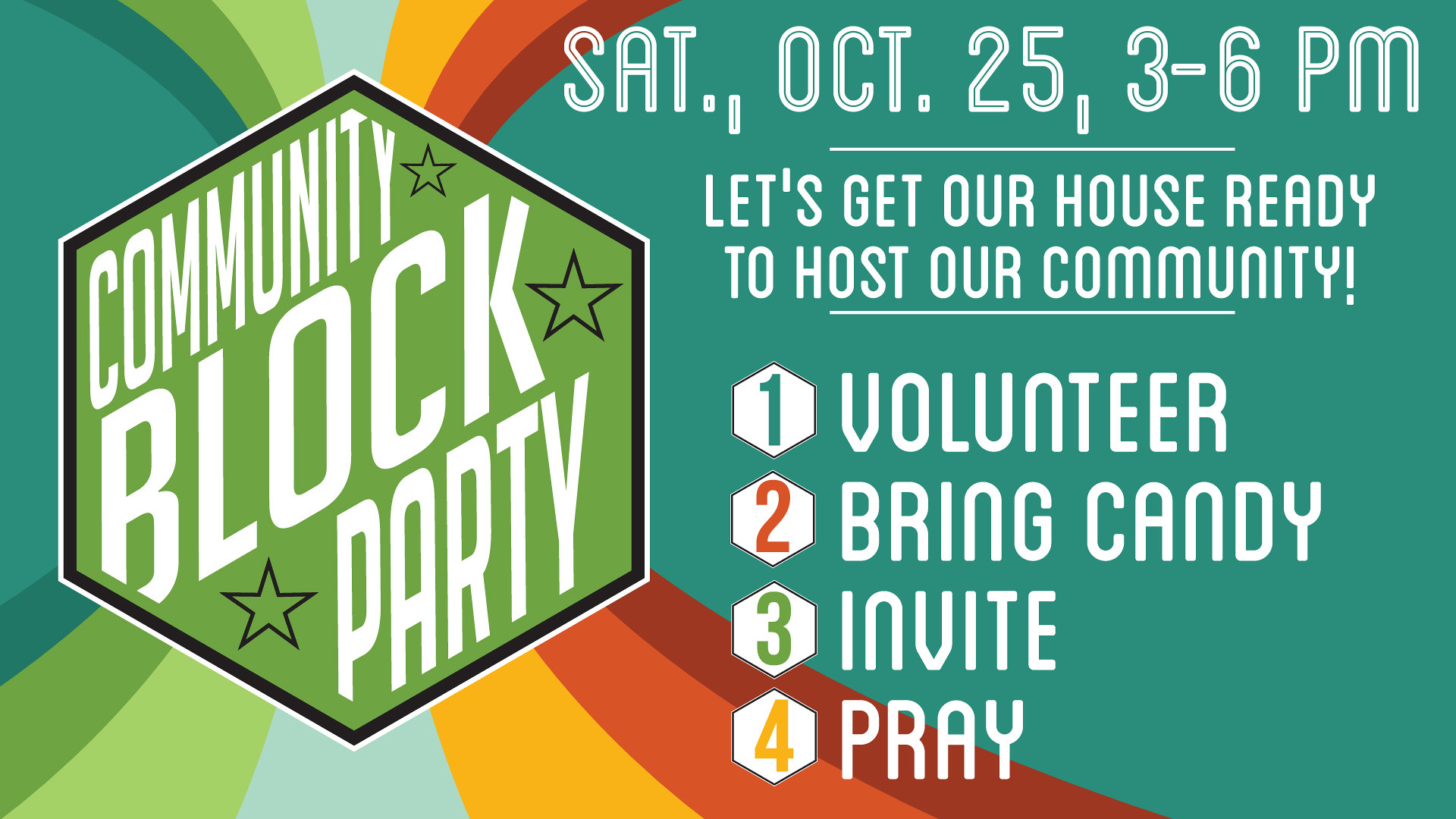This vibrant and colorful advertisement features a medium green background adorned with rainbow stripes radiating in multiple directions. Dominating the left side of the image is a lime green octagon with angular edges, emblazoned with the bold text "Community Block Party." Overlaying this background, at the top of the image, the event details are written in a white, disco-style font: "Saturday, October 25, 3 to 6 p.m." Just below, an encouraging message reads, "Let's get our house ready to host our community!" followed by an exclamation mark. Sequentially listed in varying colors, the four action items are: 1. Volunteer (green), 2. Bring candy (red), 3. Invite (green), and 4. Pray (yellow). This graphic serves as an engaging invitation and call-to-action for community members to participate actively in the upcoming event.